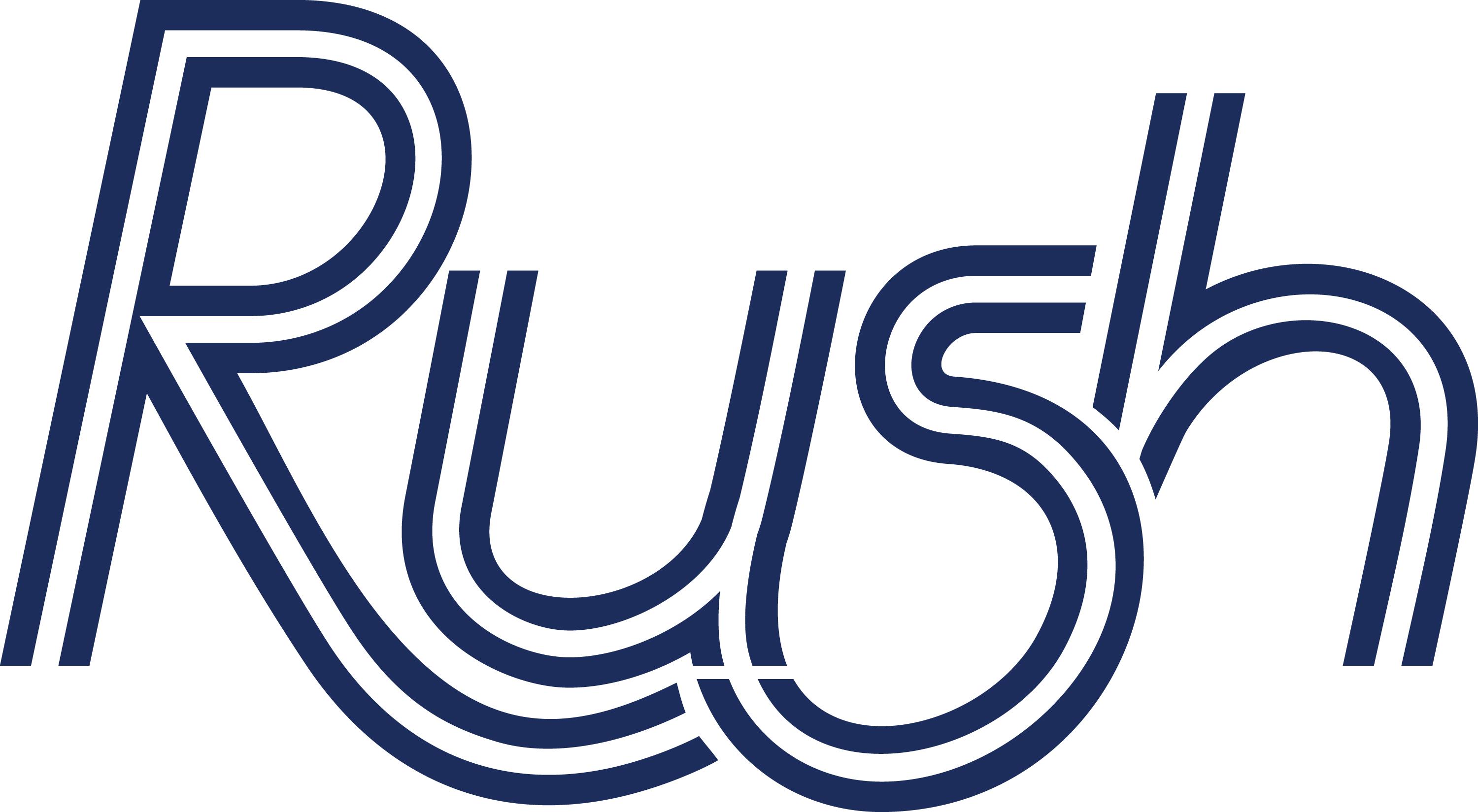The image features the word "RUSH" rendered in a highly stylized, elegant font. The letters exhibit a sophisticated interplay of color, primarily a navy blue, with white elements that create a striped effect throughout the text. The letter "R" prominently extends downward, with its elongated tail curving beneath the connected "U." The "U" seamlessly merges into the following "S," forming a continuous, fluid design. Additionally, the "H" appears to emerge from behind the "S," adding to the dynamic composition of the typography. The entire word takes center stage against an unadorned, stark white background, making it the focal point of the image.